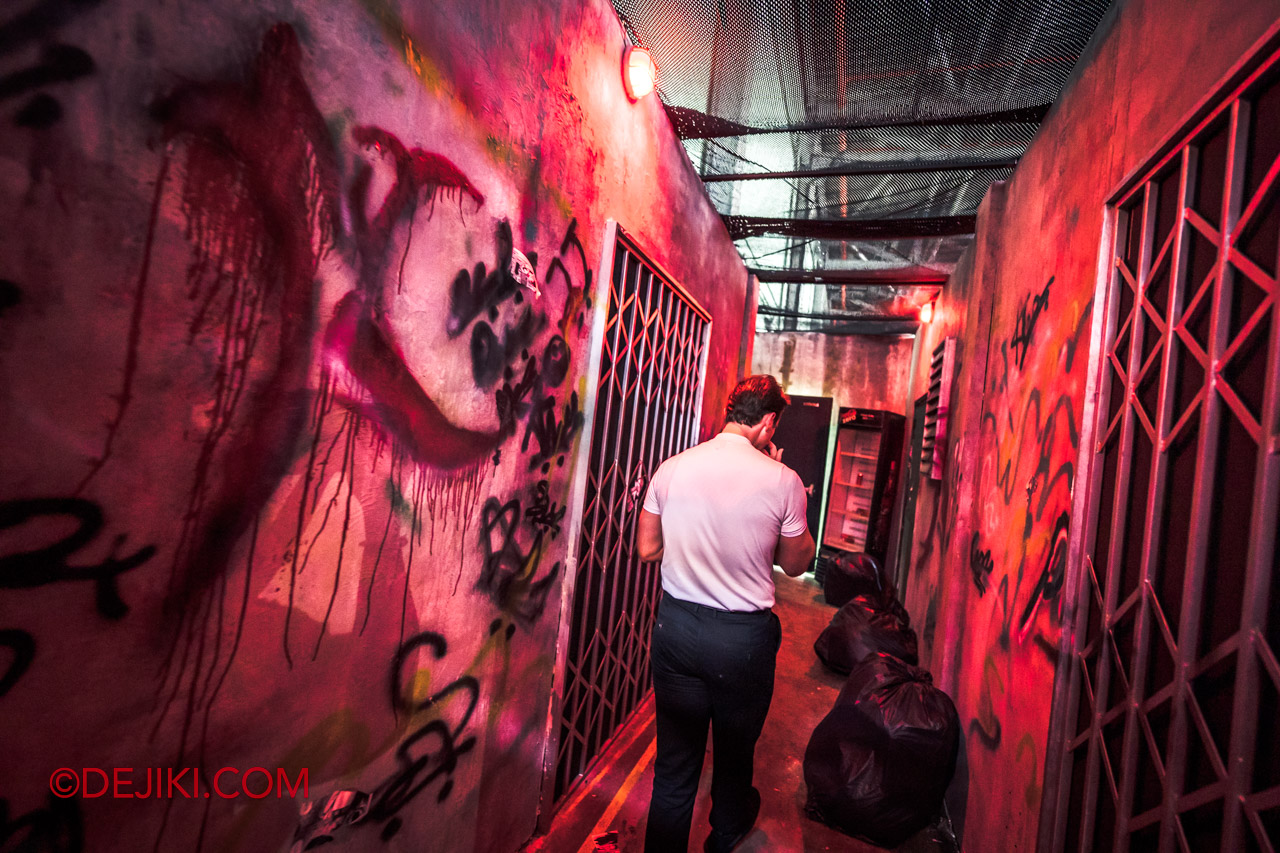In a vivid photograph dominated by a reddish hue, a man in a white polo shirt tucked into dark dress pants walks through an alleyway-like corridor. The image, taken in landscape mode, features extensive graffiti on the walls, adding a gritty atmosphere. "DEJIKI.com" is marked in the bottom left corner in red. Overhead, a black netting spans the ceiling, which appears to slope upward to the right, giving the scene a confined, almost warehouse-like feel. The corridor is lined with bags of trash on the right side, while light bulbs with a yellowish-red tint illuminate the space, one situated closer to the camera and another farther down. The man, with short brown hair, walks towards the end of the alley, where a gated area and a vending machine stand. The vending machine, positioned at the far end, seems to have a few items on four distinct shelves. Ahead, the corridor curves to the right, suggesting the pathway continues beyond the visible scene.